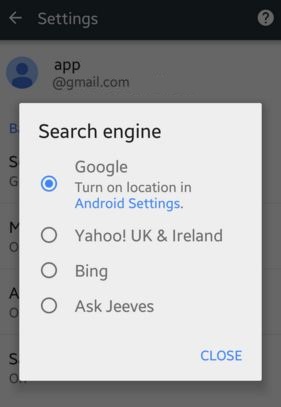A screenshot of a smartphone settings page is displayed with a prominent pop-up window in the center. The rectangular popup has a white background and is titled "Search Engine." The first option in the list reads "Google - Turn on location in Android settings," highlighted with a blue dot inside a circle, and outlined with a blue line. The text "Android settings" within this line is also colored blue. Following this, in gray text, are additional search engine options: "Yahoo UK and Ireland," "Bing," and "Ask Jeeves." Each of these alternatives is unmarked. In the lower right-hand corner of the popup, the word "CLOSE" is written in all capital letters and blue print, indicating an option to exit the popup.